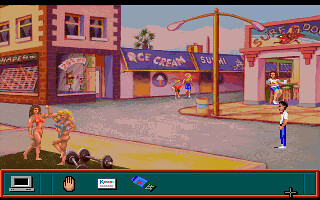A small screenshot captures a vintage video game, reminiscent of a classic handheld or old Atari NES title. The scene depicts a bustling downtown area adjacent to a beach, where a boardwalk atmosphere is evoked. A lone character is positioned in the middle of the street, donning blue pants, a white shirt, and a red bow tie. Prominent details enhance the nostalgic feel: in the bottom left corner, two women in bikinis, appearing to be weightlifters, are caught mid-high-five with barbells scattered at their feet. In the background, an ice cream shop invites patrons, while a small restaurant named Surf Dogs is visible to the right, adding to the overall beach town charm. No recognizable game details are provided in the image.